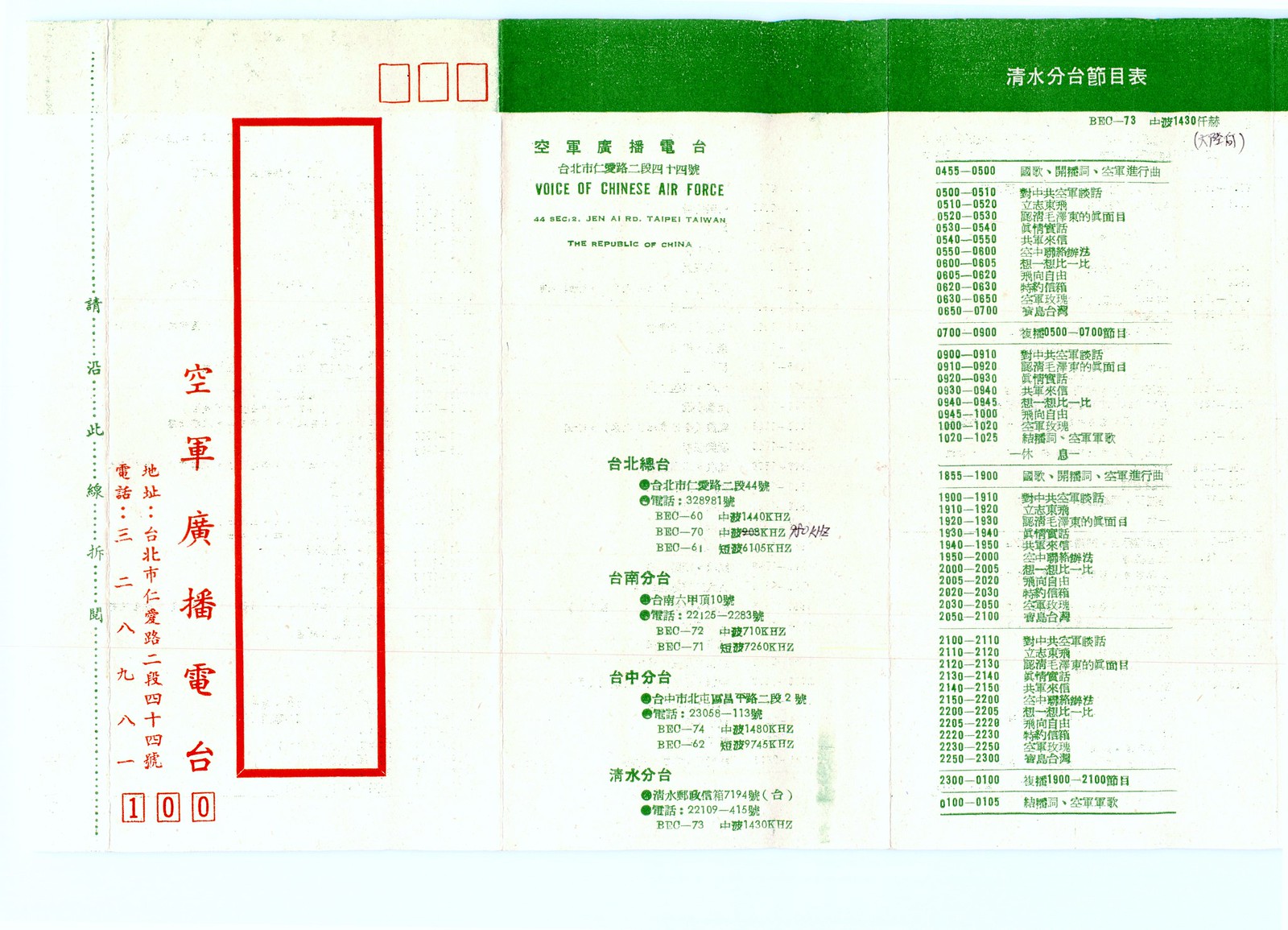The image is of a document, possibly a card, associated with the Chinese Air Force, titled "Voice of Chinese Air Force, the Republic of China." The text is predominantly in Mandarin and Chinese characters. The left part of the document features red text on a white background, with a prominent red rectangle at the bottom containing the number 100, and a large red triangle with three red squares above it. There are Chinese characters adjacent to these shapes. The right side of the document is largely green and white, with four vertical sections of Chinese text interspersed with numerical sequences such as 3289181, 60, 70, and 61. There's also a green banner at the top of this section. The document is divided into two main panels - left with red and white, and right with green and white - each containing structured columns of text and numbers. A potential stamp feature is visible on the left side, contributing to its official and detailed presentation.